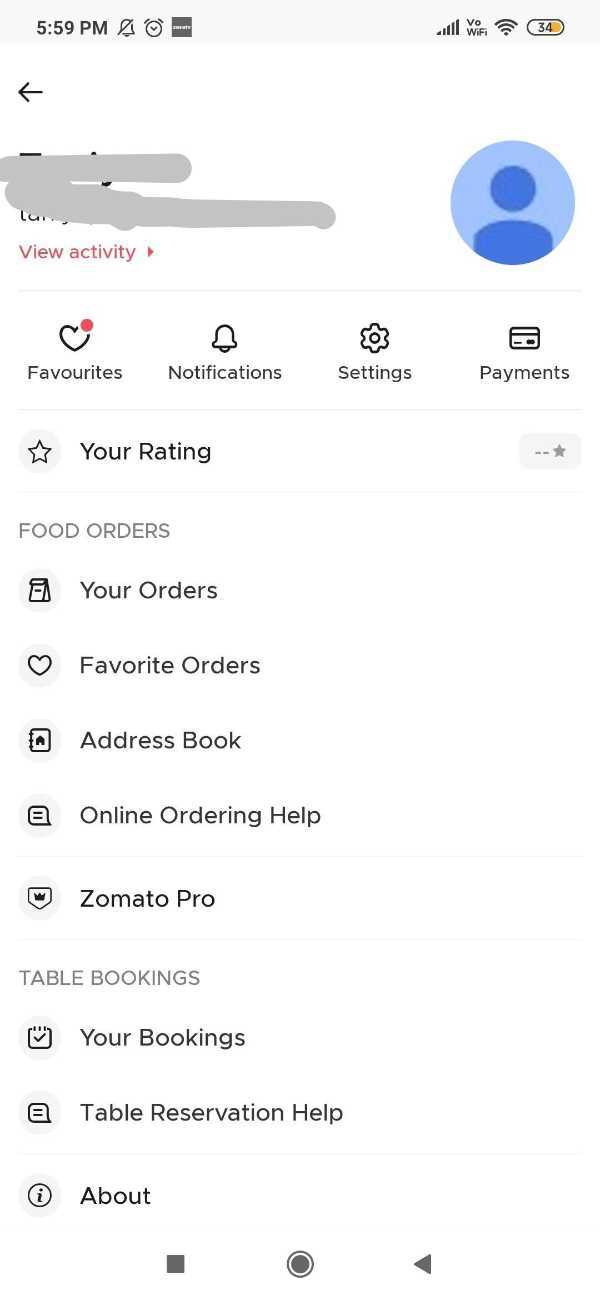A screenshot captured from a smartphone displaying a food ordering app interface. The time shown on the screen is 8:59. At the top left, there's a back arrow, with an alarm clock icon below it. A gray scratched-out section is present, possibly concealing sensitive information. Beneath this, the options "View Activity" and "Read" are listed, followed by a username icon depicted as a blue picture.

The main interface features sections labeled "Favorites," "Notification Settings," and "Payments." There's a star icon indicating user ratings, which is currently blank or shows a dash meaning no ratings yet. 

On the left side, a menu includes "Your Orders," "Favorite Orders," "Address Book," "Online Ordering," and "Help." A label displaying "Model Pro" appears as well. In a separate section titled "Table Bookings," options for "Your Bookings," "Table Reservation Help," and "About" are provided.

At the very bottom of the screen, a black square is seen. The middle features a circular dot, encircled, next to a triangle pointing to the right. This implies that the app offers functionalities such as viewing past orders, managing reservations, and handling payments.